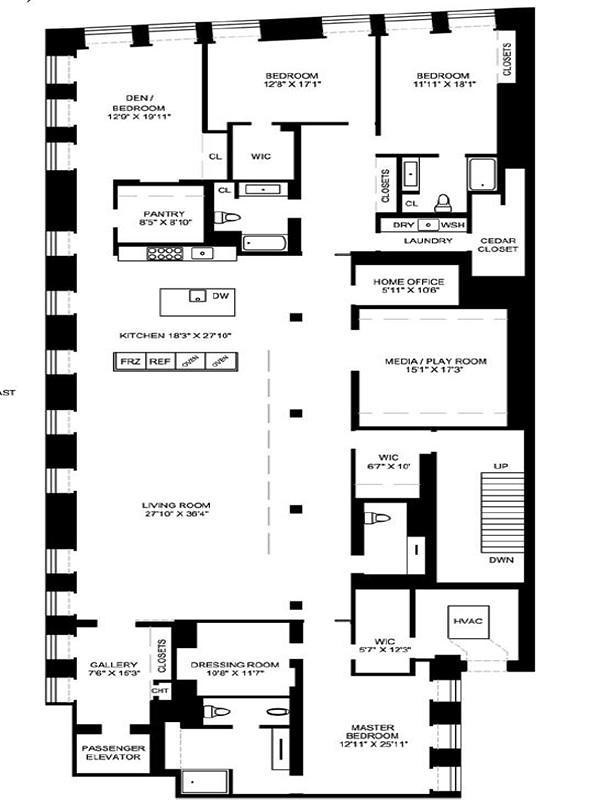The image depicts a detailed floor plan of a residential apartment. The layout is a square-ish shape, divided into various sections with specified dimensions. 

At the very top left of the plan is a den/bedroom, which measures 12 feet by 19 feet, 11 inches. Adjacent to this room on the top is another bedroom, sized at 12 feet, 8 inches by 17 feet, 1 inch. To the right of this bedroom is yet another bedroom measuring 11 feet, 11 inches by 18 feet, 1 inch, with a closet on its right side.

Proceeding downward, there's a bathroom outfitted with a sink, a toilet, and a bathtub. Continuing along, there is a hallway that houses the laundry area with a dryer and washer, leading to a cedar closet. 

To the upper left of the den/bedroom is a closet, next to which lies a pantry measuring 8 feet, 5 inches by 8 feet, 10 inches. Below this pantry, there is a kitchen, which is 18 feet, 3 inches by 27 feet, 10 inches, equipped with a refrigerator, freezer, and oven. Further down the plan, there's a spacious living room, measuring 27 feet, 10 inches by 36 feet, 10.4 inches.

In the bottom left corner, there is a gallery area, 7 feet, 6 inches by 15 feet, 3 inches. Next to it, extending towards the right, is a dressing room, measuring 19 feet, 8 inches by 11 feet, 7 inches. This leads to a bathroom connected to the master bedroom located at the bottom-right corner of the plan, which measures 12 feet, 11 inches by 25 feet, 11 inches.

Further up, there is a water closet measuring 5 feet, 7 inches by 12 feet, 3 inches, adjacent to the HVAC (heating, ventilation, and air conditioning) unit connected to the outside. On the upper side of the plan, a media/playroom measuring 17 feet, 3 inches connects to a home office above it, which measures 5 feet, 11 inches by 10 feet, 6 inches.

Overall, the floor plan includes bathrooms, closets, a kitchen, a hallway, living areas, and other essential spaces, carefully laid out to provide a clear overview of the apartment's layout and dimensions.